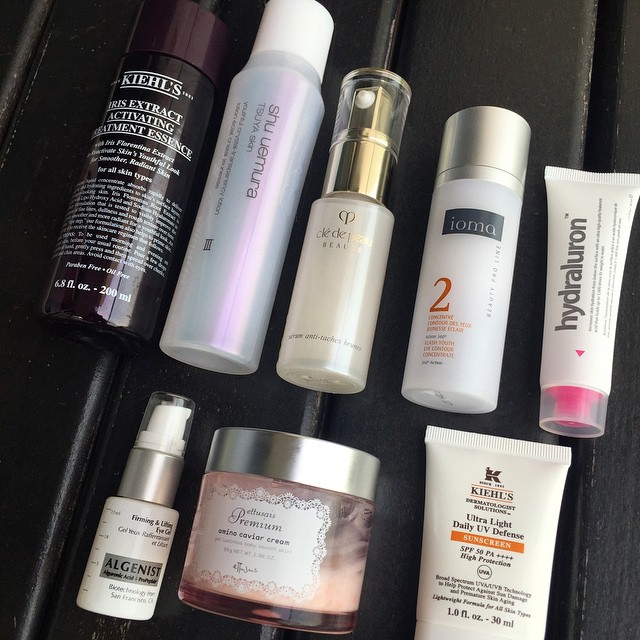The image showcases an array of beauty products arranged on a black wooden surface. At the bottom, partially cut off, there is a bottle of Kiehl's Ultra Light Daily UV Defense sunscreen, identifiable by its white packaging with black and orange accents. 

Moving up to the middle of the image, we encounter a jar of Premium Amino Caviar Cream, featuring a silver lid and an intricate lacy logo, the cream inside presenting a pinkish hue. Adjacent to this is a firming and lifting eye gel from Algenist, distinguished by its white and silver design and topped with a white cap.

In the upper section, all the bottles are tilted at an angle. Starting from the top left, there is a black bottle of Kiehl's Activating Treatment Essence, marked with its capacity of 6.8 fl oz (200 ml). Next to it is a plastic bottle with a white cap labeled Shu Uemura, with the text oriented sideways. Further along is a gold-accented bottle, seemingly a perfume or beauty product labeled DD something beauty. 

Following this, there is a white bottle from IOMA with the number 2 in orange text, featuring a silver cap and a logo overlaid on a textured black design. Lastly, towards the middle right of the image, there is a white tube with a clear cap (pink on the inside), labeled Hydraluron, complete with a trademark symbol (TM).